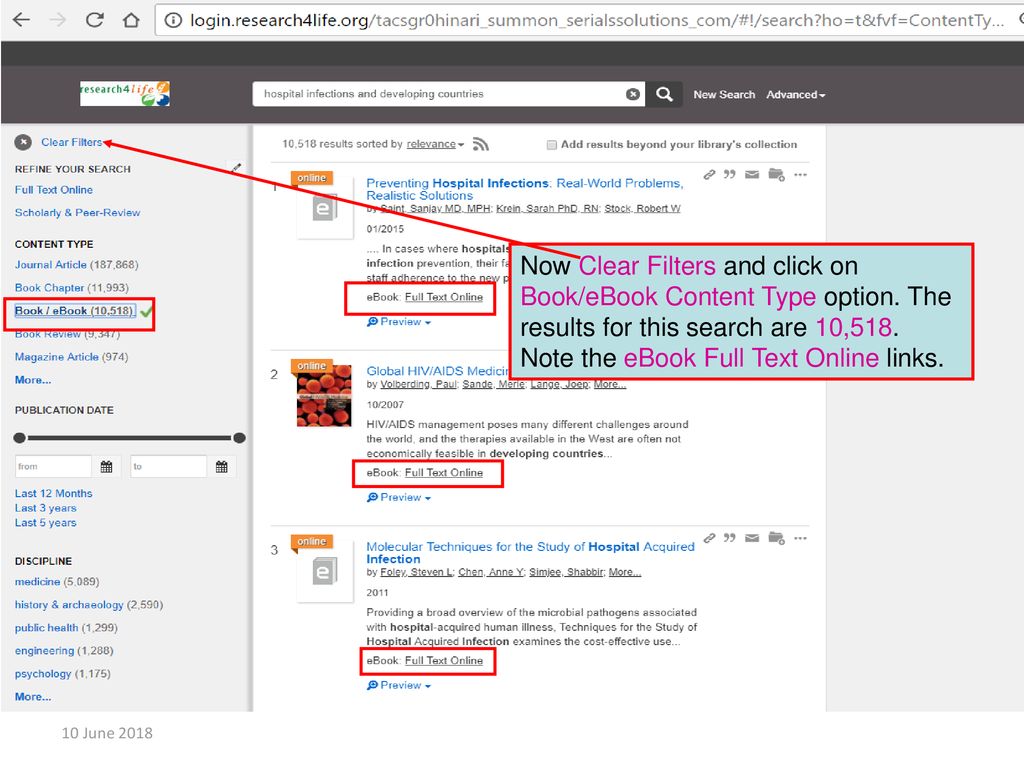The image depicts a screenshot of an online search on an older or specialized browser displayed on a computer screen. The search bar shows the URL "login.researchforlife.org/..." followed by an obscured string. The banner at the top contains an input field where the search query "hospital infections in developing countries" has been entered. The browser includes a dated stamp, "10 June 2018," near the bottom left, indicating when the search was conducted or when the browser interface was captured.

The interface seems to be an illustration or tutorial of the search engine rather than an active search by the user. This is evidenced by instructional elements such as a hyperlinked "Clear Filters" text in blue at the top left, accompanied by a red arrow from a teal box with a red outline, prompting users with "Now Clear Filters" in purple. Below this, users are directed to click on "Book/Ebook" under the content type, highlighted in magenta, with other instructional texts in black.

The search results display a significant number, "10,518," in purple, indicating the number of results found for the query. Additionally, multiple elements in the search results are highlighted with red rectangles, directing attention to the "Ebook Full Text Online" links. More red rectangles emphasize selections under content types, showcasing "Book/Ebook" on the left sidebar and several instances within the search results.